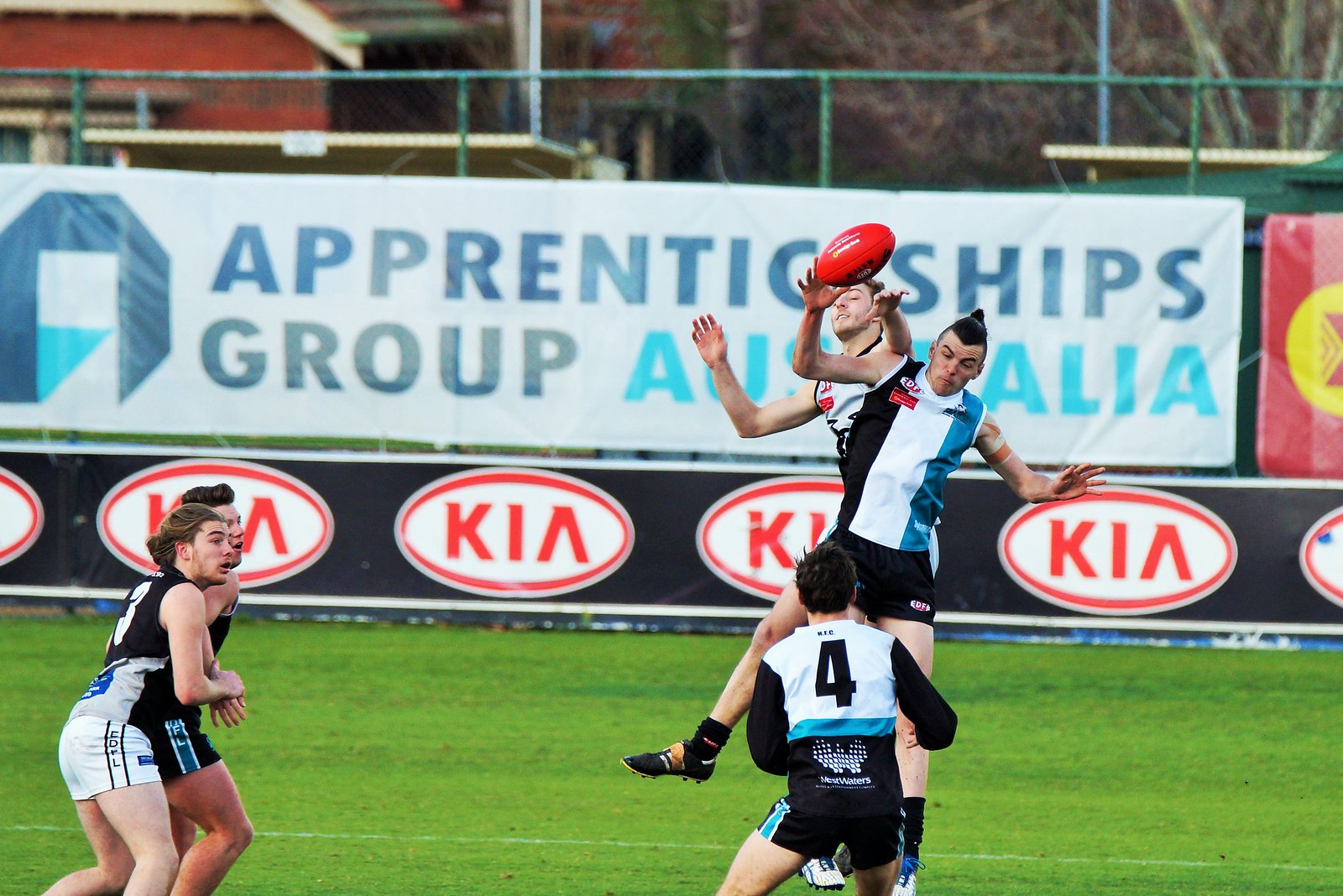This image captures a dynamic moment in a live rugby match on a vibrant green grass field. Two teams are in action: one team is clad in black, gray, and white jerseys, while the other dons black, blue, and white kits. At the heart of the scene, a player sporting a black, white, and blue striped shirt leaps into the air, reaching for a red and black rugby ball. Opposite him, another player jumps in pursuit of the ball, both contributing to the intense atmosphere. The background features a green chain-link fence, a prominent "Apprenticeships Group Australia" banner, and repetitive red and white Kia logos on a black border along the edge of the field. Beyond the fence, a brick building and some dry trees add to the outdoor stadium's setting, encapsulating the essence and energy of the rugby game in Australia.